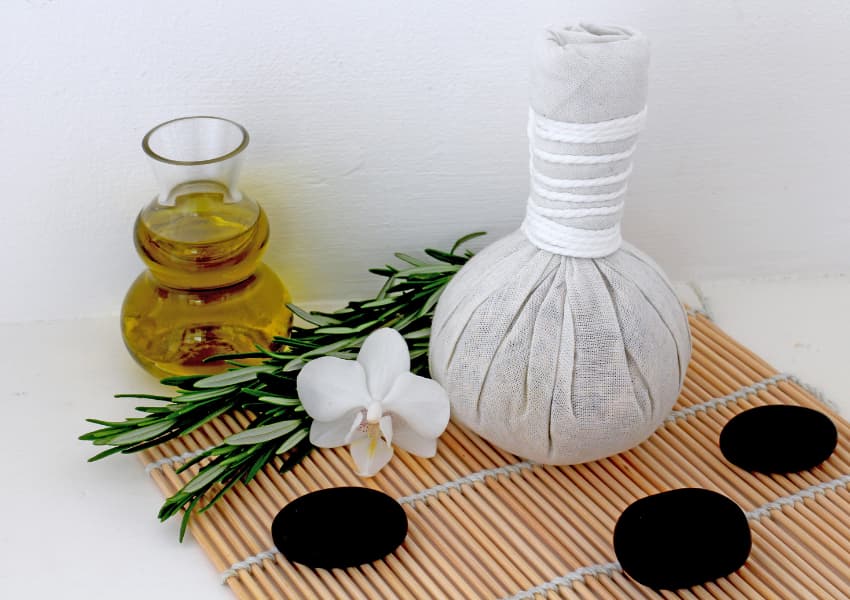This close-up photo captures a white countertop or shelf attached to a subtly textured white wall in the background. Centrally arranged on a light bamboo mat, three black coasters scatter around a striking white flower and bright green flower stems. Dominating the middle of the scene, a vase-like object is wrapped tightly in a rough white cloth with white string around its neck, almost resembling a gourd in shape. To the back left, just off the mat, an open glass container—about two-thirds filled with a honey-colored liquid—sits, with its double circular design and open top hinting at its function, like that of a flask or olive oil bottle.